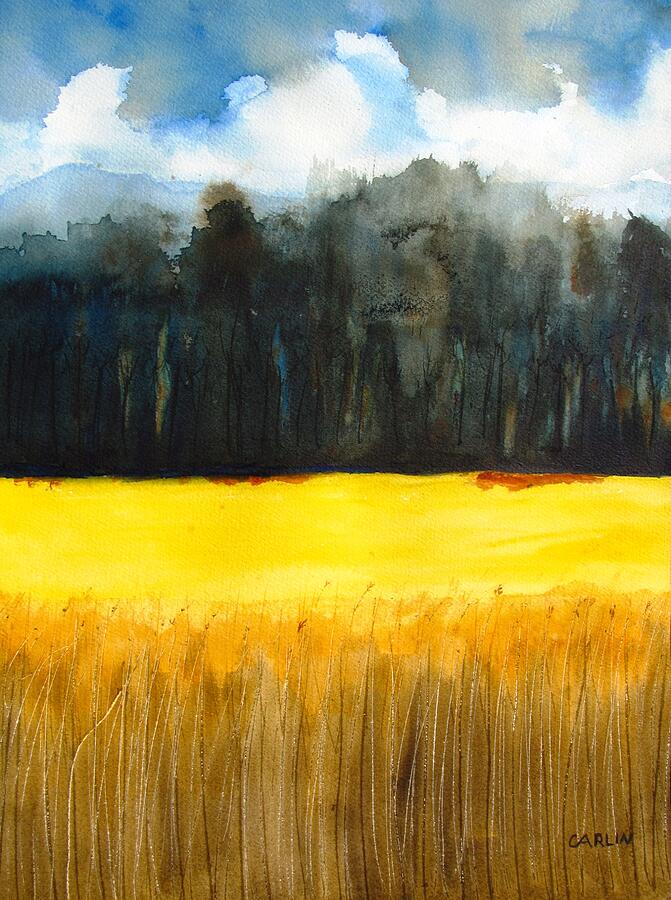This vivid, abstract watercolor painting by an artist named either Carlin or Garlin features a striking and impressionistic landscape. The foreground is dominated by a field of tall, wheat-like grasses in a range of bright yellows, with some upward-reaching stalks topped with puffy yellow flowers. This yellow expanse extends halfway up the image, transitioning abruptly into a dark blue-black and green area that likely represents a forest at the edge of the field. Farther in the distance, the scene lightens into whiter blues and whites, suggesting rolling hills or a distant mountain range, beneath a blue sky dotted with white clouds. The entire image, characterized by its out-of-focus style and vibrant blending of colors, carries a watermark of the artist's name in the bottom right corner, aligning the viewer's eye with the artwork's layered depth and intricate details.